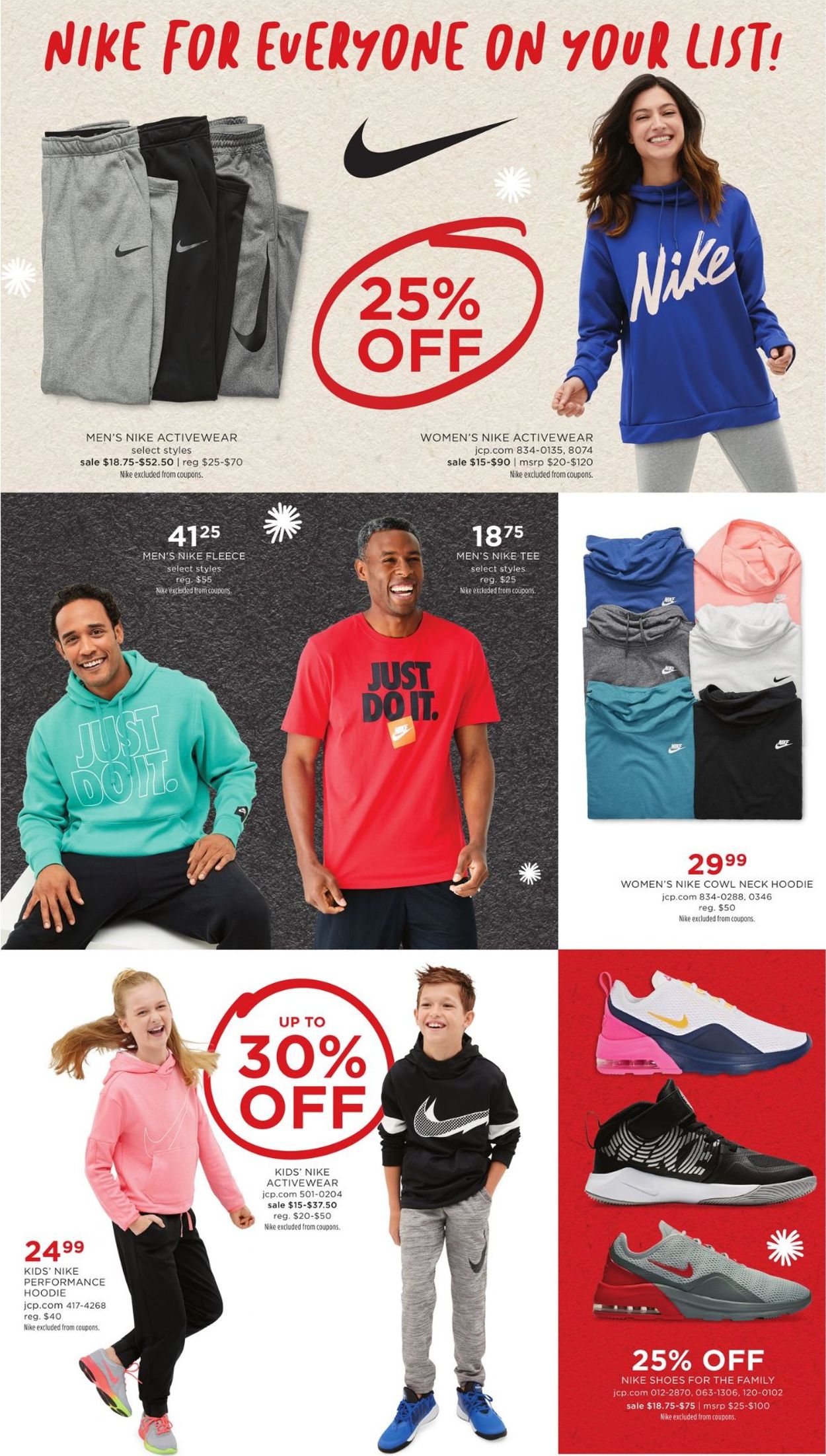The image features a top section with a light purple box displaying a promotional message in red text: "Nike for everyone on your list". A bold, black Nike swoosh is prominently shown along with a red circular emblem indicating a 25% discount. On the left side, three pairs of pants are displayed, each marked 25% off. To the right, a woman is shown modeling a blue Nike long-sleeve shirt, which is also 25% off.

Below this, against a black background, there are several items listed with specific prices: a green hoodie priced at $41.25, a red "Just Do It" t-shirt priced at $18.75, and women's Nike hoodies priced at $29.99.

At the bottom of the image, on a white background, a "Up to 30% off" offer is highlighted inside a circle. Next to this, a young boy and girl are seen wearing hoodies, each priced at $24.99. Adjacent to them, a red box showcases three different pairs of shoes, all offered at a 25% discount.